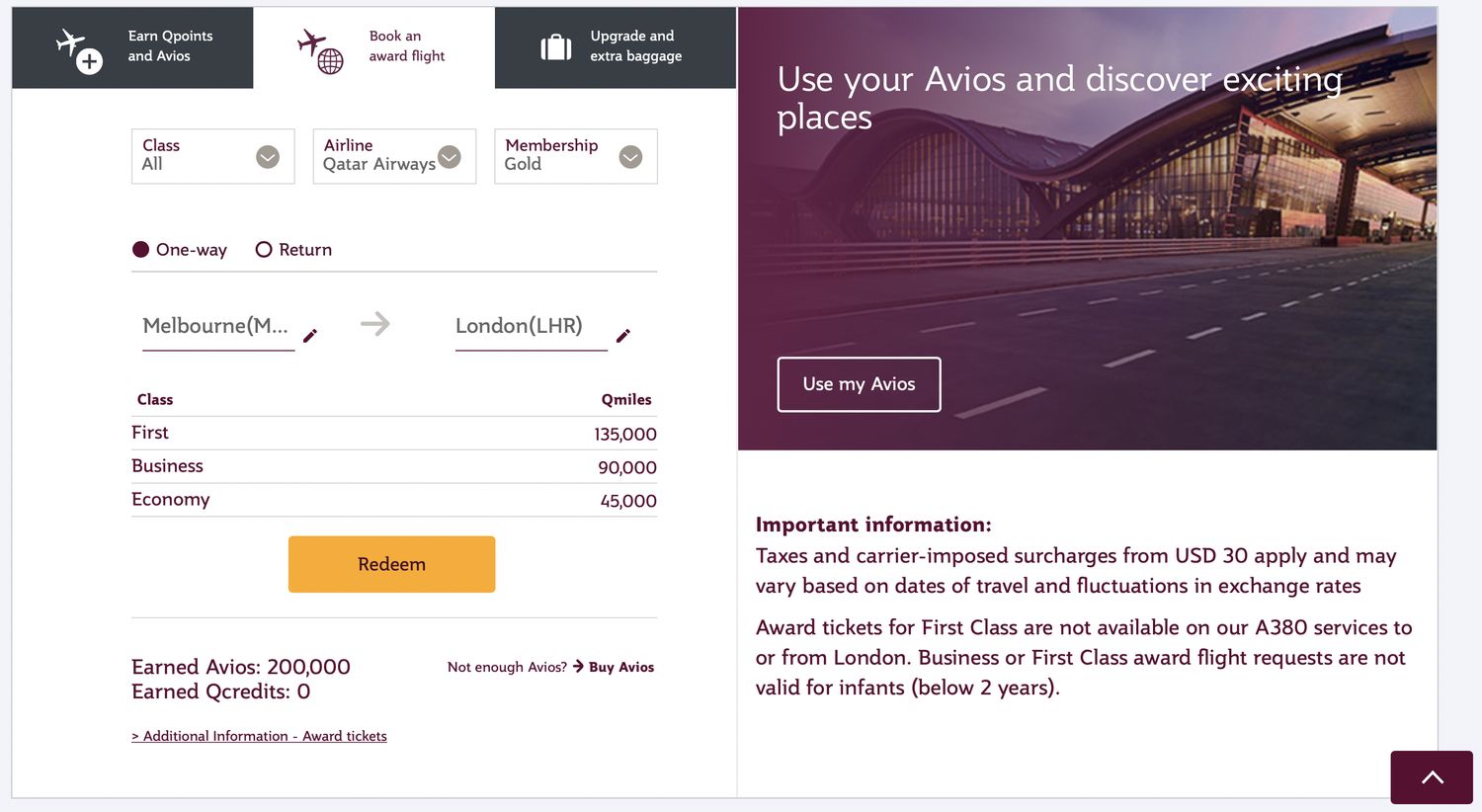**Detailed Caption:**

The image pertains to aviation travel. In the top left corner, three primary categories are displayed: "Earn Points and Avios," "Book an Award Flight," which is currently selected and highlighted in purple, and "Upgrade and Extra Baggage" to the right. 

Below these categories, there are three selection boxes. The first box is labeled "Class" with "All" beneath it. The second box reads "Airline" with "Cater Airways" beneath it. The third box is titled "Membership" and shows "Gold" beneath it.

Further down, there are options for "One Way" and "Return," each accompanied by a selectable circle to their left.

To the right of these options, a large image featuring an airplane runway is displayed. The image bears the text "Use your Avios and discover exciting places." 

At the bottom left, a rectangular button says "Use My Avios." Below this button, there is an important note that reads "Important Information: Taxes and carrier-imposed surcharges start from USD 30 and may vary based on dates of travel and fluctuations."